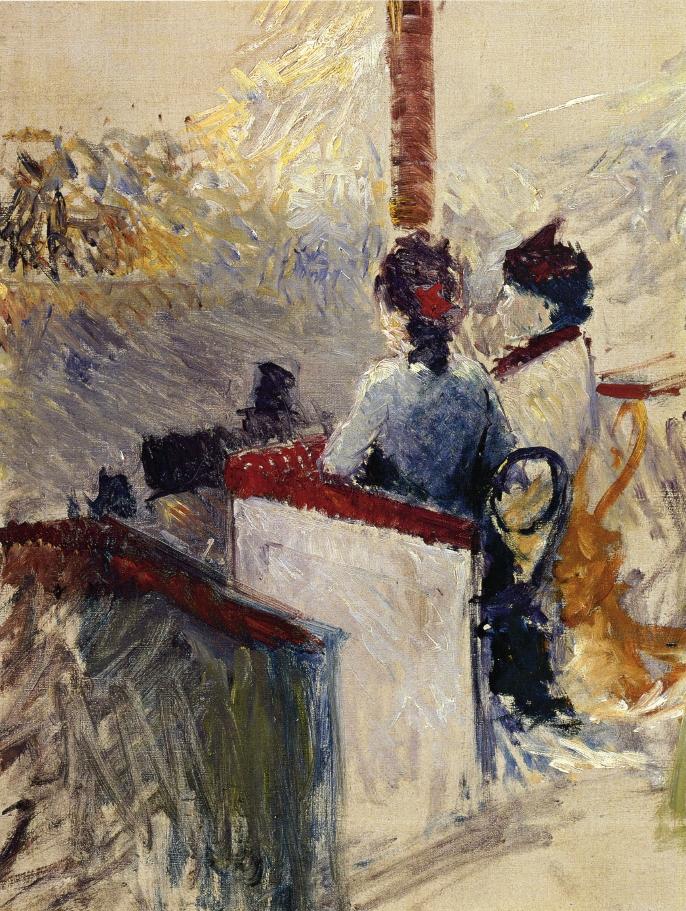The painting depicted in the image evokes an Impressionist style reminiscent of artists like Van Gogh or Monet, characterized by detailed and textured paint strokes. The scene features the backs of two women seated in a booth that appears to be part of a larger setting—possibly a play or some form of scenic lookout. Both women have their hair up, adorned with noticeable red ribbons, and are dressed in clothing with touches of blue, white, and maroon trim. Despite the painting's somewhat ambiguous details, the vivid use of color, including predominant reds, whites, and dark shades, creates a rich and lively composition. The booth itself is white with a reddish maroon trim. While specific elements like mountains or other figures are not clearly defined due to the impressionistic style, the textured layers and the apparent roughness of the paint add a distinct, tactile depth to the scene. The overall artwork invites curiosity and further exploration into its detailed yet elusive imagery.